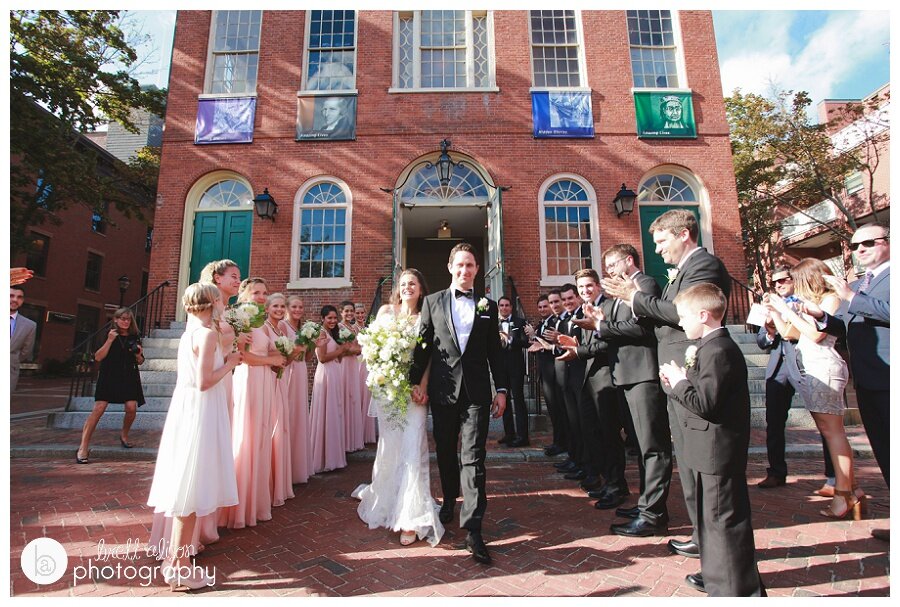In this vibrant color photograph, a joyous wedding procession unfolds against the backdrop of a stately brick building, possibly a rustic courthouse or a modest chapel. At the forefront, the bride and groom, clad in stunning attire, walk hand in hand, basking in the sunny day's light and occasional shadow. The bride dazzles in her elegant white gown, her hands tenderly holding a bouquet of white flowers. Surrounding them, the wedding party assembles in complementary colors: bridesmaids in charming pink dresses and groomsmen in sharp black tuxedos. A young boy and girl also join the assemblage, adding a touch of innocence to the scene. The entire group, numbering around twenty, captures the momentous occasion with lively expressions of celebration. Below the image, white text bears the watermark of an unreadable photography credit, preserving the joyful memory of the day.